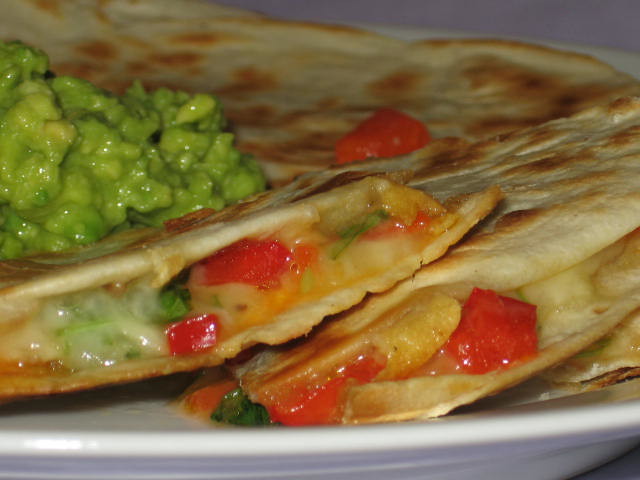The close-up image showcases a Mexican dish featuring several cheese quesadillas stacked on a white ceramic plate, with the dish’s edge just visible at the bottom of the frame. The tortillas are a tan color with golden brown spots and crispy dark edges, indicating they have been fried to perfection. Each quesadilla reveals a melty interior filled with a mix of orange and white cheeses, chopped tomatoes, red peppers, chicken chunks, and possibly lettuce. A generous, chunky scoop of guacamole with a slightly grainy texture sits atop the uppermost quesadilla, its light green and yellow hues adding contrast. Adjacent to the guacamole on the left side of the image is a small wedge of tomato, enhancing the vibrant and appetizing presentation.